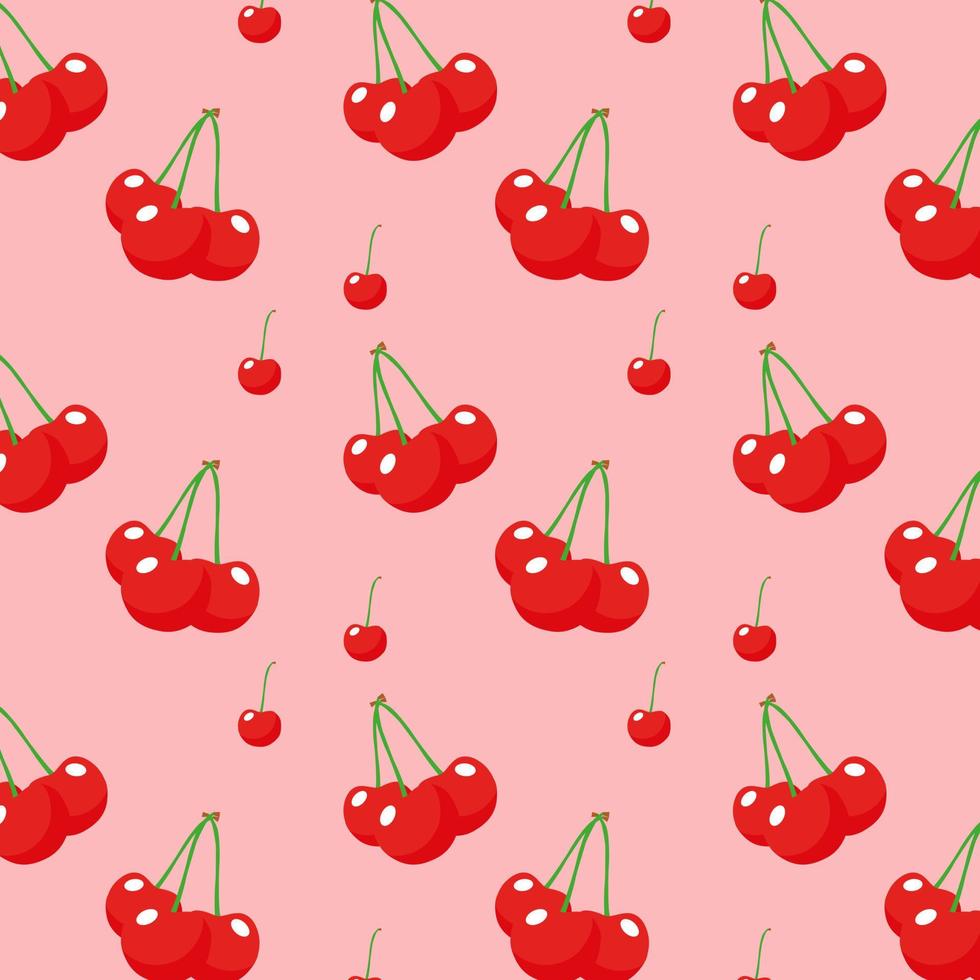The image features a pink, wallpaper-like design adorned with a repeating pattern of cherries. There are two types of cherry illustrations: clusters of three cherries and single cherries. The clusters show three cherries with the middle one slightly in front of the other two, all connected by thin green stems that converge and are tied together with a little ribbon at the top. There are eighteen such clusters arranged in three diagonal lines, with each cluster and single cherry angled differently—some pointing to the right, others to the left. In between these clusters, individual bright red cherries with white reflective spots are scattered, each also featuring a green stem. This alternating pattern of cluster, single, cluster, single, creates a structured yet dynamic visual over the pale pink background.